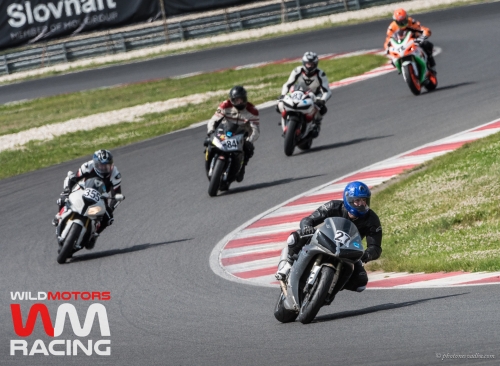The photograph captures an intense motorcycle race on a tarmac track with five motorcycles engaged in the heat of competition. In the forefront, a blue motorcycle bearing the number 27, ridden by a motorcyclist in a blue helmet, black jacket, and silver boots, is seen turning a corner. Close behind, a white motorcycle labeled with the number 35, piloted by a racer clad in a white jacket, black and white helmet, white pants, and white boots, follows diligently. The winding track, forming an S-shape, is bordered by distinct white and red stripes on both sides. Lush green grass flanks the track, with a gravel pit visible on the left side. An inscription in white and red text, "Wild Motors WM Racing," is prominently watermarked in the bottom left corner. Each rider’s helmet color - ranging from blue to orange - complements their corresponding motorcycle, painting a vivid picture of synchrony and speed.